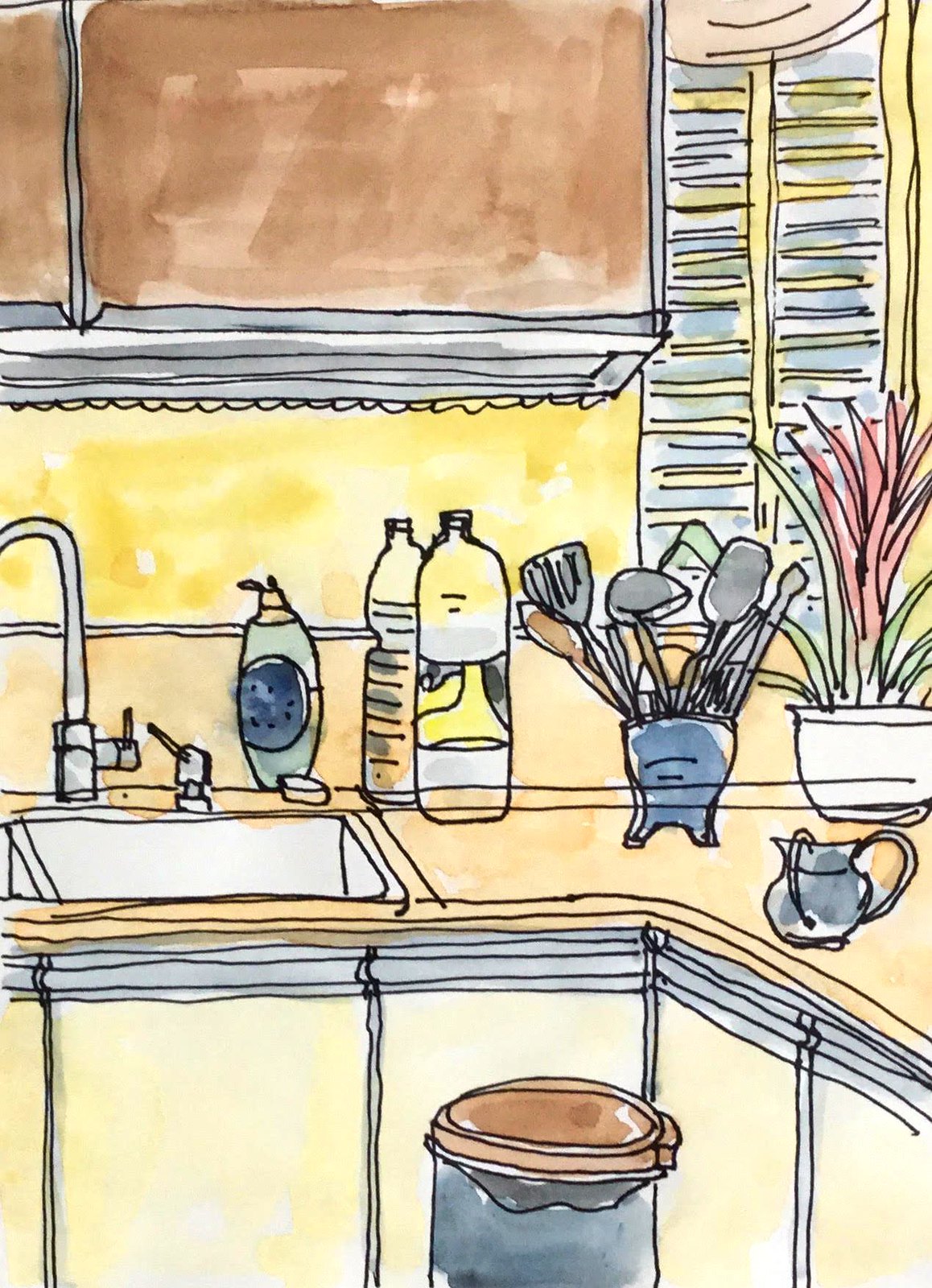This animated kitchen setting features a detailed arrangement of various elements. At the very bottom stands a trash can with a gray body and a brown lid. In front of the trash can, the lower cabinets are highlighted in a whitish-tan color, with contrasting gray tops. Above these cabinets lies a light orange-brown countertop, with a sink positioned on the left side. The sink and its accompanying faucets are depicted in light gray tones.

To the right of the sink, a dish soap bottle stands, characterized by a light gray hue, a bluish circle, and a light brown cap. Adjacent to the dish soap are two additional bottles, followed by a collection of gray kitchen utensils neatly arranged in a light blue container. Further to the right, a house plant in pink and gray hues adds a touch of vibrancy.

Above the countertop, a blue windowsill frames a window, while a yellow backsplash extends to the left. Topping off the scene, the lower parts of the upper cabinets are shown in gray and brown shades, completing this meticulously detailed, animated kitchen environment.